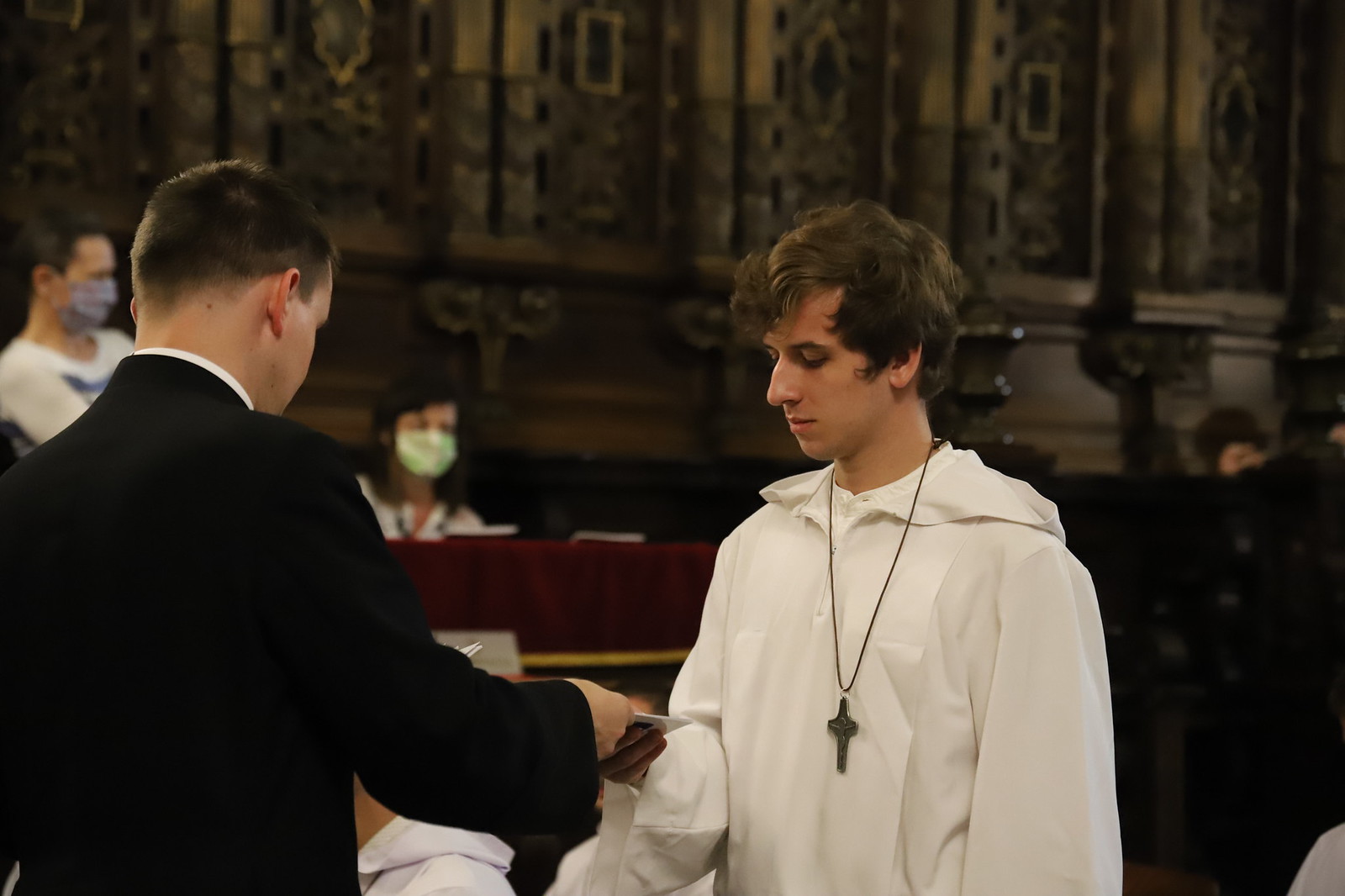In this detailed photograph taken inside a grand, ornately decorated cathedral, two figures are prominently featured in the foreground. The gentleman on the left, wearing a black suit with a white collar, has short brown hair and is handing an envelope to the man on the right. The recipient, a young man with wavy brown hair, is dressed in a white robe with a hood resting on his back. A cross necklace hangs around his neck. The backdrop consists of highly decorated walls with intricate filigree and textures, including ornate marble and wooden carvings. Red velvet benches line the church interior, and several masked churchgoers are seen seated in the background, indicating that this image might have been taken during the COVID-19 pandemic. The overall scene suggests a solemn, religious ceremony.